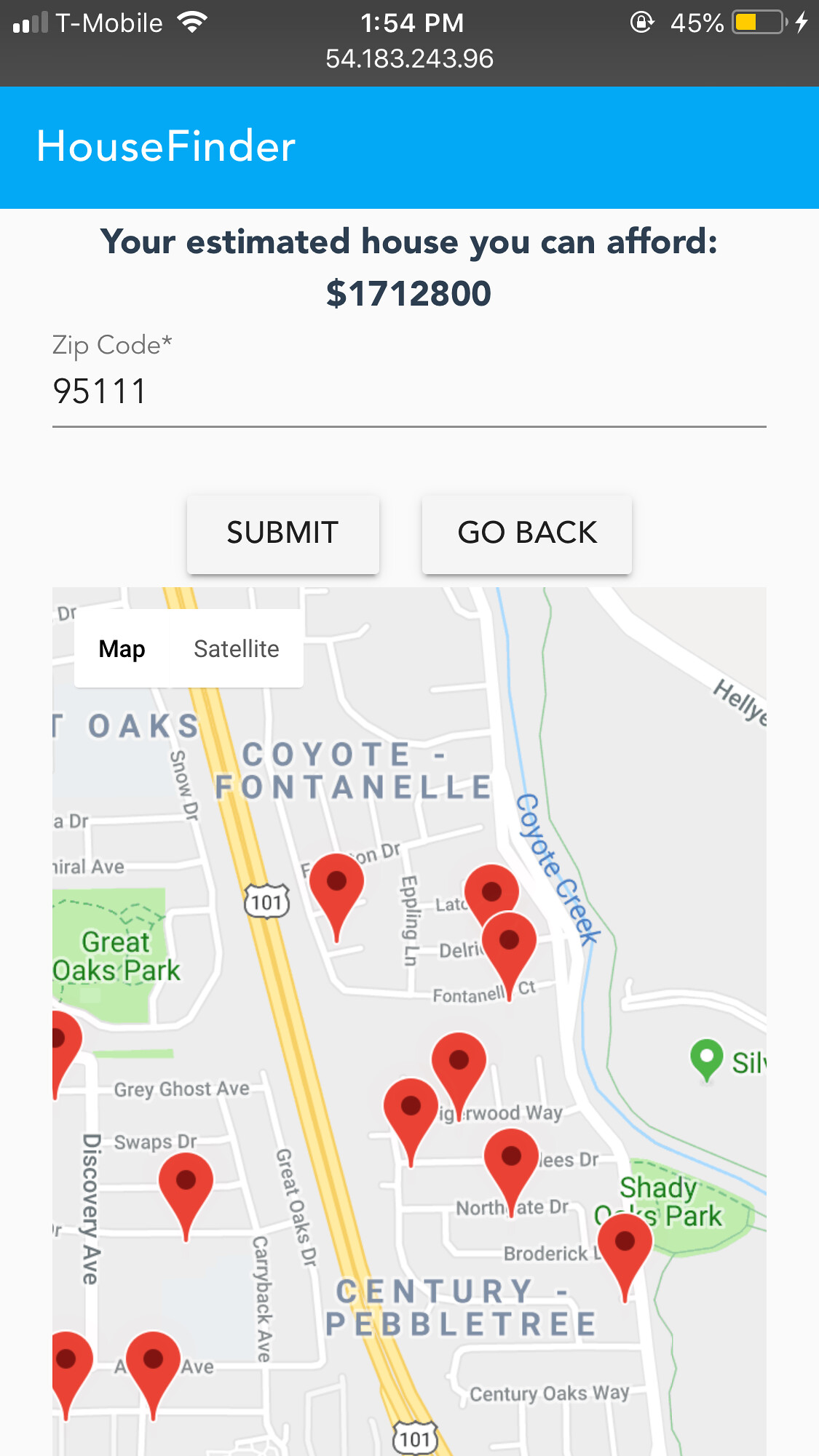This is a screenshot taken on a T-Mobile phone, exhibiting various status indicators at the top, including the number of signal bars, the T-Mobile carrier label, Wi-Fi symbol, the time (1:54 p.m.), GPS coordinates, battery percentage (45%), and battery icon. The screenshot was captured within an app called House Finder, displaying a large, bold title reading "Your Estimated House You Can Afford" followed by the amount "$1,712,800." Below this information, the zip code 75111 is specified.

Two buttons, "SUBMIT" and "GO BACK," are prominently featured underneath the financial estimate. These buttons are outlined in gray and contain capitalized black text. Below the buttons, the screenshot reveals a detailed map highlighting the areas of Coyote, Fontenelle, Century Pebble Tree, and a yellow-highlighted highway labeled 101. The map also demarcates parks in green and a water body, Coyote Creek, in blue. Various streets criss-cross the screen, adorned with red pinpoints potentially indicating different house locations.

The app's title, House Finder, is displayed in white font against a blue background stretching across the top row, giving the interface a clean and structured look.